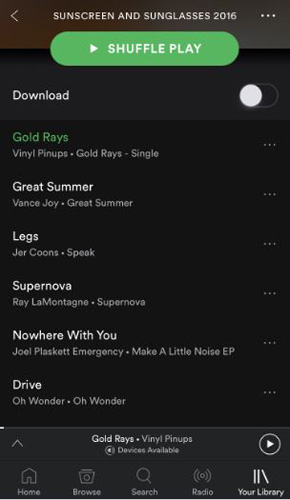The image depicts a music application interface, characterized by a sleek, user-friendly design. The background is predominantly black, with white text and vivid green highlights that accentuate key elements. At the very top of the screen, the title "Sunscreen and Sunglasses, 2016" is prominently displayed. To the upper left, a return arrow symbol and a caret icon are visible, providing navigation options. Directly beneath the title, a prominent green button labeled "Shuffle Play" invites users to mix up the playlist.

A downloadable button or link is situated near the shuffle play option. The playlist showcases a collection of summer-themed tracks, starting with "Gold Rays" by Vinyl Pinups, followed by "Great Summer" by Vance Joy, "Legs" by Jerichoons, "Supernova" by Ray Montague, "Nowhere With You" by Jewel Plaskett Emergency, and "Drive" by Oh Wonder.

Beneath the tracklist, a progress bar allows users to track their listening progress, accompanied by a play button for easy control. At the bottom of the interface, a set of icons provides quick access to essential features: Home, Browse, Search, Radio, and Your Library. This intuitive layout ensures a seamless musical experience for the user.